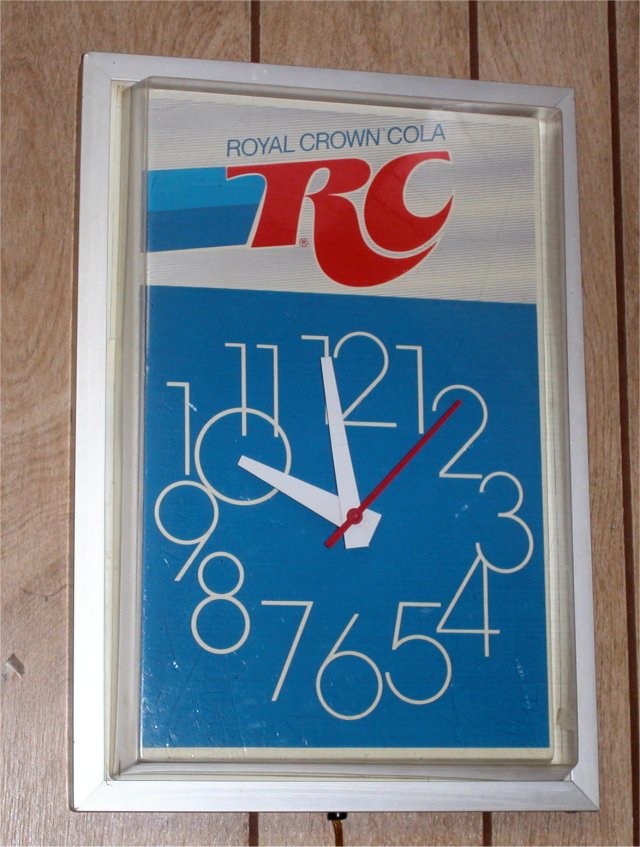The image features a vertically oriented rectangular clock with a white border and a clear, enclosed face. At its center, there is a blue square clock displaying white numerals. The clock is equipped with thick white hour and minute hands, along with a red second hand. Above the clock face, the text "Royal Crown Cola" is prominently displayed in blue, followed by the stylized red cursive initials "RC." Adjacent to this, on the left, are vertical stripes in light and dark blue colors. The clock appears to be constructed out of plastic and shows signs of wear, including minor dings and fading on its face. It is mounted against a wood-paneled wall that is light brown with darker stripes accentuating the individual panels.